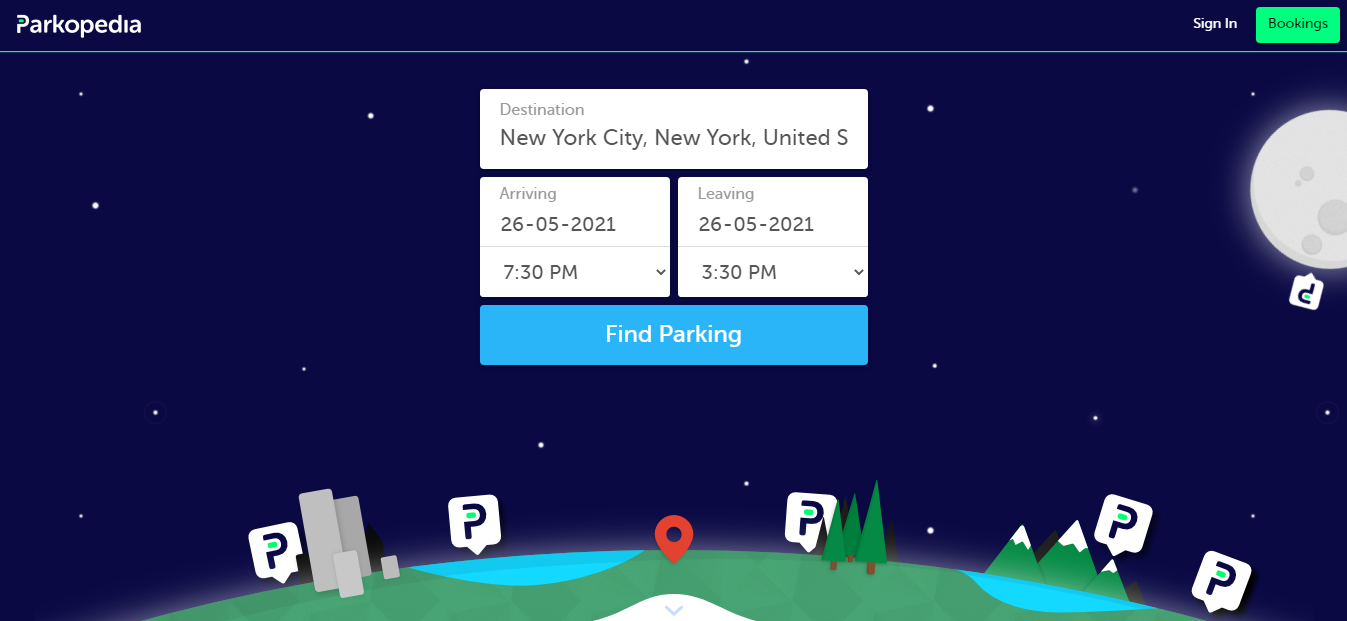The image depicts a webpage from Parkopedia, a minimalist and user-friendly platform designed to help users find parking spots. The interface prominently features a search bar labeled "Enter a destination," where someone has input "New York City." The arrival and departure details are specified as arriving on May 26, 2021, at 7:30 p.m., and leaving on the same day at 3:30 p.m. This discrepancy in the timeline suggests an error, as traveling back in time is not feasible.

Below the search bar is a large, blue "Find Parking" button intended to help users locate available parking spots in the specified area, useful given New York City's notorious parking difficulties. At the top of the page, the Parkopedia logo is visible on the left, while sign-in and bookings buttons are positioned on the right, indicating options for reserving parking spots or managing existing reservations. Adding a whimsical touch, a cartoony, computer-generated image of Earth from space decorates the page, accentuating the site’s global reach and accessibility.